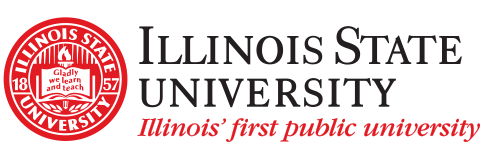The image features a pristine letterhead design from Illinois State University. Dominating the top portion, "ILLINOIS STATE UNIVERSITY" is prominently displayed in bold, black, all-capitalized, and elegant typography. Directly beneath it, in a smaller, red, and equally ornate font, the phrase "Illinois's first public university" is delicately inscribed, lending a scripted and sophisticated touch.

To the left of the main heading, a striking emblem stands out. This mostly red logo is encircled by two concentric white outlines. Encircling the top half of the logo in black printed letters are the words "Illinois State University," while the bottom half reads "University" with the establishment date, "1857," split with '18' on the left side and '57' on the right.

Central to the emblem is an open book, illustrating the motto "Gladly We Learn and Teach" within its pages. The book is illuminated by a torch with a vibrant flame, symbolizing knowledge and enlightenment. Surrounding the book, vertical lines extend upward, while wheat-like images are nestled below, adding to the emblem's agricultural symbolism.

The overall design is minimalist yet sharp, focusing solely on the university's identity and historical elements without any additional information, reflecting a polished and professional aesthetic reminiscent of an official letterhead.